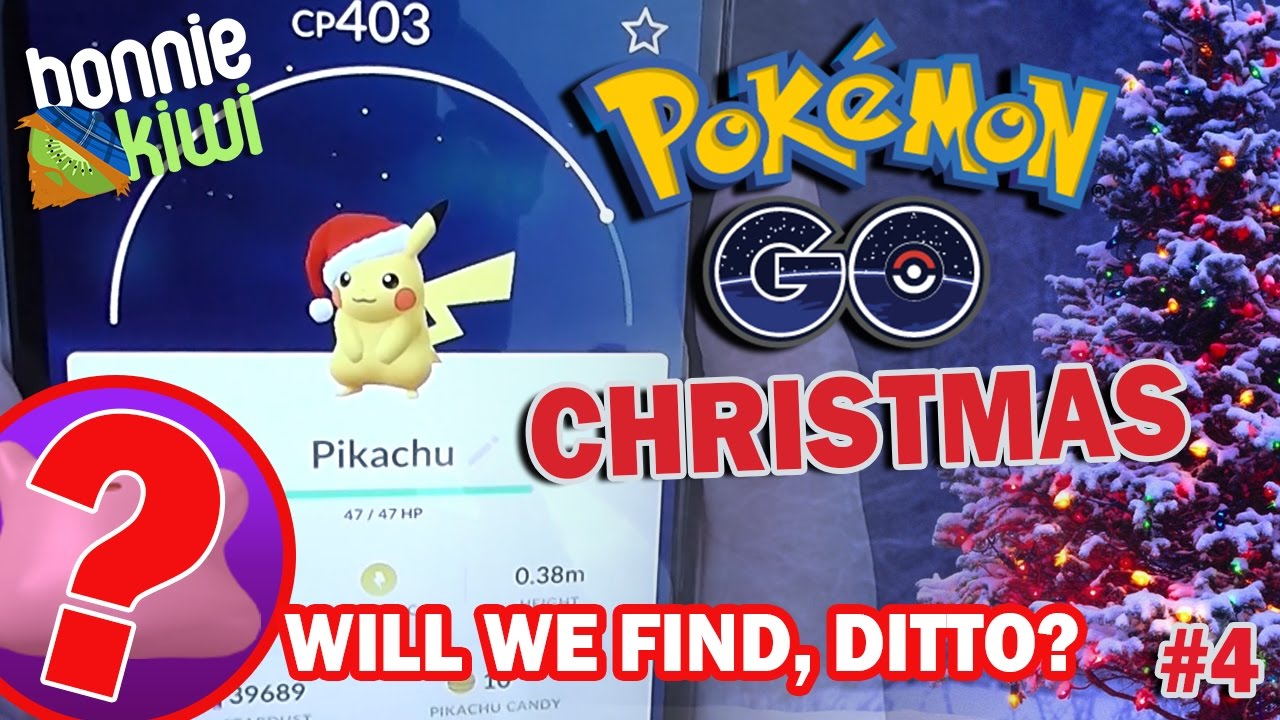This image depicts a Pokémon Go Christmas advertisement featuring a characteristically festive Pikachu. Positioned slightly off-center to the left, the rosy-cheeked, yellow Pikachu is donning a charming Santa hat. Below Pikachu, the text indicates his name, "Pikachu," along with his stats, "47/47 HP" and "0.38 M." Overlaying the statistics paper are words that read, "Will we find Ditto?" giving a sense of anticipation.

In the bottom corners, various textual elements are present: the lower right corner features "#4," and the lower left corner includes an image with a red question mark overlay. Subtly framing the scene on the right side of the background is a beautifully decorated Christmas tree, illuminated by twinkling lights that are gently muted by a layering of freshly fallen snow on the branches and bulbs.

At the top of the image, the text "CP 403" is accompanied by the name "Bonnie Kiwi," and a vibrant white star is prominently featured above the Pokémon. This enchanting holiday-themed advertisement melds the whimsical world of Pokémon with the cozy, magical spirit of the Christmas season.